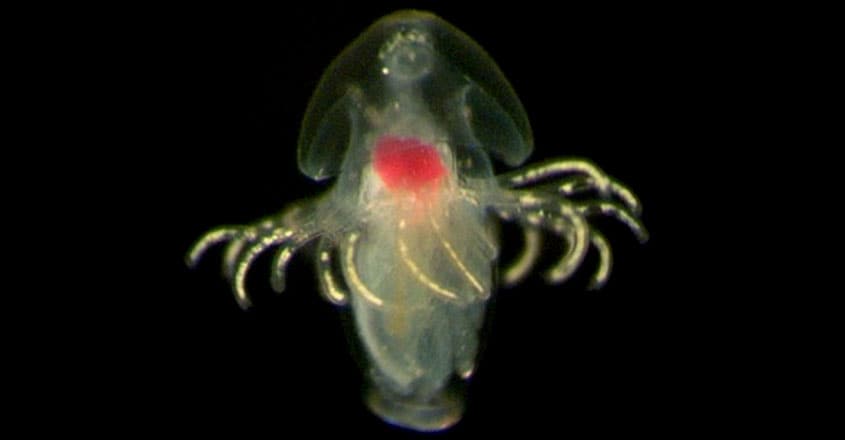In this image, a translucent, jellyfish-like creature is centered against a stark black background, giving it an ethereal, almost glowing appearance. The creature has a mushroom-shaped head that is clear and curved, allowing a glimpse of an eye-like structure near its top. Inside its transparent body, there appears to be a red, heart-shaped blob, hinting at internal organs. From its midsection, a ring of tentacles, numbering roughly around 12-14, extends outward in various directions. The base of the body transitions into a cylindrical shape, resembling the figure of a person draped in a dress, adding to its exotic, otherworldly look.